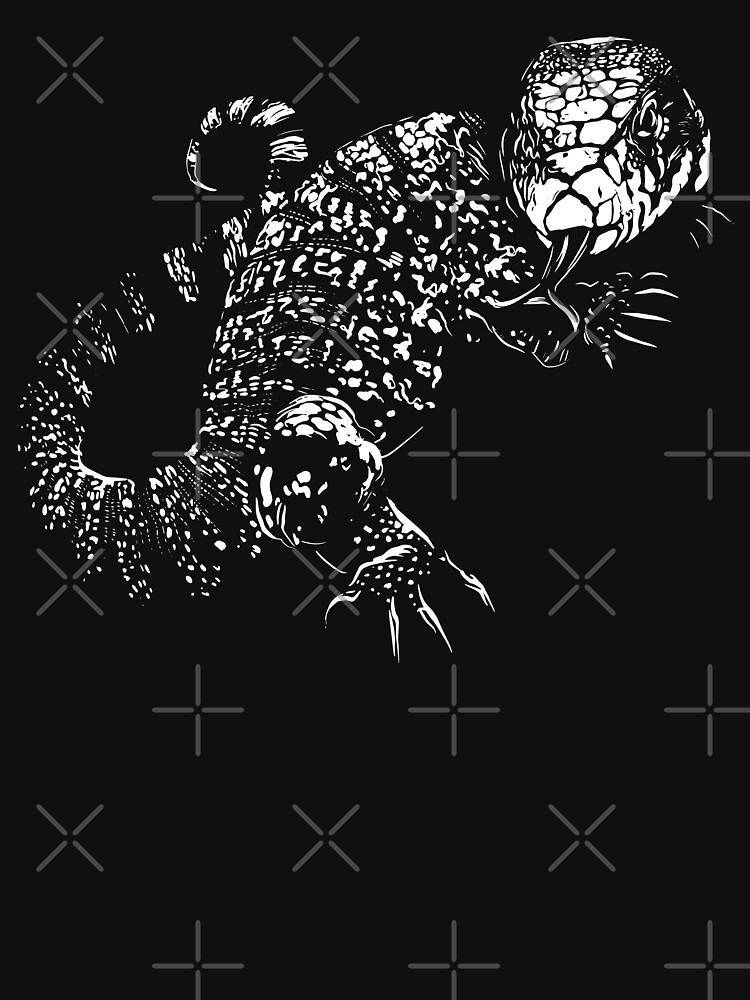The image presents a striking black and white depiction of a lizard-like creature against a stark black background adorned with a grid pattern of light gray crosses and Xs. The lizard, appearing semi-transparent with intricate white dot patterns and markings, dominates the scene from the middle to the upper portion of the frame. Its menacing posture is highlighted by a forked tongue slithering out of its mouth, long claws, and a coiled tail, giving the impression it is emerging from the background with a three-dimensional effect. The lizard's face is the clearest detail, conveying a sense of eerie intensity as it seemingly stares directly at the viewer. The overall dark and somewhat spooky appearance is enhanced by the contrasting light reflections on the lizard's scales and skin.